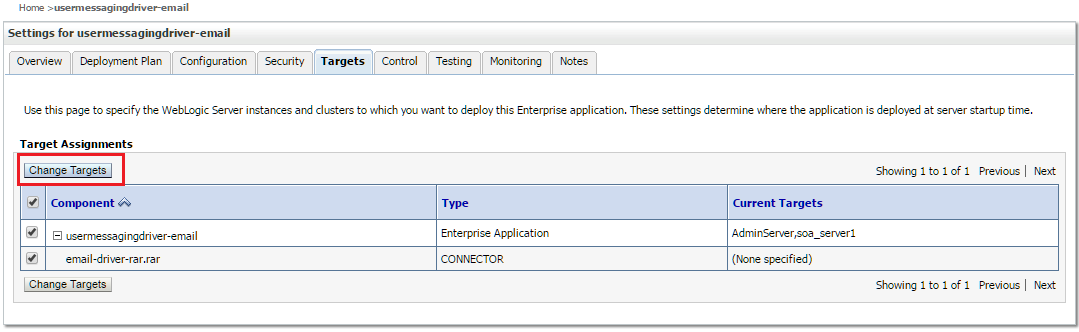The homepage section displayed is dedicated to managing the "User Messaging Driver - Email" settings. At the top of the header, the section title "Settings for User Messaging Driver - Email" is prominently featured.

Beneath the header, a series of horizontal tabs spans from left to right, labeled as follows: Overview, Deployment Plan, Configuration, Security, Targets (currently selected), Control, Testing, Monitoring, and Notes.

The primary content area includes text that instructs the user, reading: "Use this page to specify the WebLogic Server instance and clusters to which you want to deploy this enterprise application. These settings determine where the application is deployed at server setup time."

In bold black text, the subtitle "Target Assignments" is displayed, accompanied by a red box labeled "Change Targets." To the right, control buttons labeled "Showing 1 of 1," "Previous," and "Next" are available for navigation.

A table beneath this text details the components, including their type and current targets, each with a checkbox to the left for selection:
1. **User Messaging Driver - Email:** Type: Enterprise Application; Current Targets: Admin Server, SOA_Server1.
2. **Email Driver:** File: email-driver-rar.rar; Type: Connected; Current Targets: Not Specified.

Below the table, there is an additional box for altering target assignments, along with repeated navigation controls to the right, labeled "Showing 1 of 1," "Previous," and "Next."